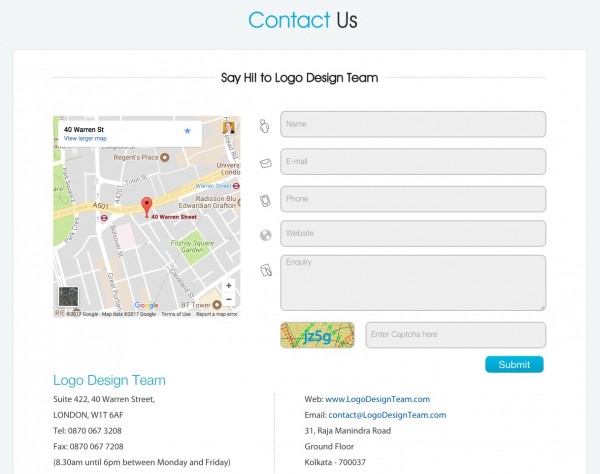In the provided image, we have a detailed map, prominently featuring a location marked by a red pin at 41st Street. The top right corner of the image displays 'Regent's Place'. The map background is predominantly grey, with various streets and landmarks highlighted, including A501, 1st Street, Madison Blvd, Edwardian, Crafton, and Square Garden.

Overlaid on the map, there is an input form located to the right of the image, with fields labeled Name, Email, Website, and Inquiry. Below these fields, there's a CAPTCHA entry labeled 'JZ5G' followed by a 'Submit' button.

In the bottom left corner of the image, the contact details for the Logo Design Team are provided, which include:
- Address: Suite 422, 41st Street, London
- Phone: 08700673208
- Fax: 08700673208
- Office Hours: 8.30am - 6pm, Monday to Friday
- Website: www.logodesignteam.com
- Email: contact@logodesignteam.com

Additionally, there is another address listed: 31st Rajah, Mananjaro, Ground Floor, Kolkata, 700037.

The overall background of the page is white, while the left and right borders are grey.